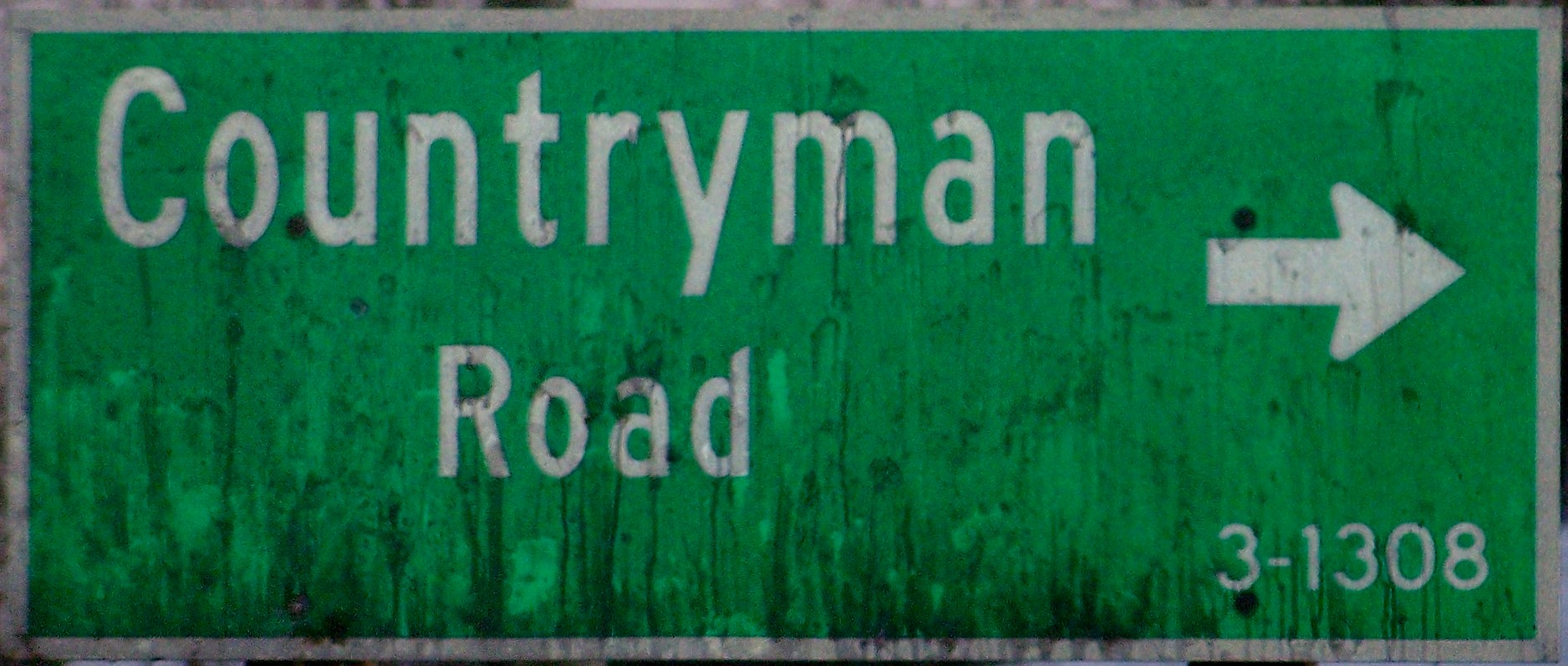This is a detailed close-up photograph of a rectangular metal street sign. The sign has a bright green background with a white reflective border. In bold white reflective lettering, it reads "Countryman Road," and features a white arrow pointing to the right. Beneath the arrow is the smaller print, "3-1308." The sign is visibly worn, with streaks of black muck and debris evident across its surface, likely from weathering and exposure to the elements. The sign is mounted using four screws visible in the image, indicating it is fixed to posts. The close-up nature of the shot highlights the dirt and wear on the sign, suggesting it is an actual real sign rather than a new or unused one.